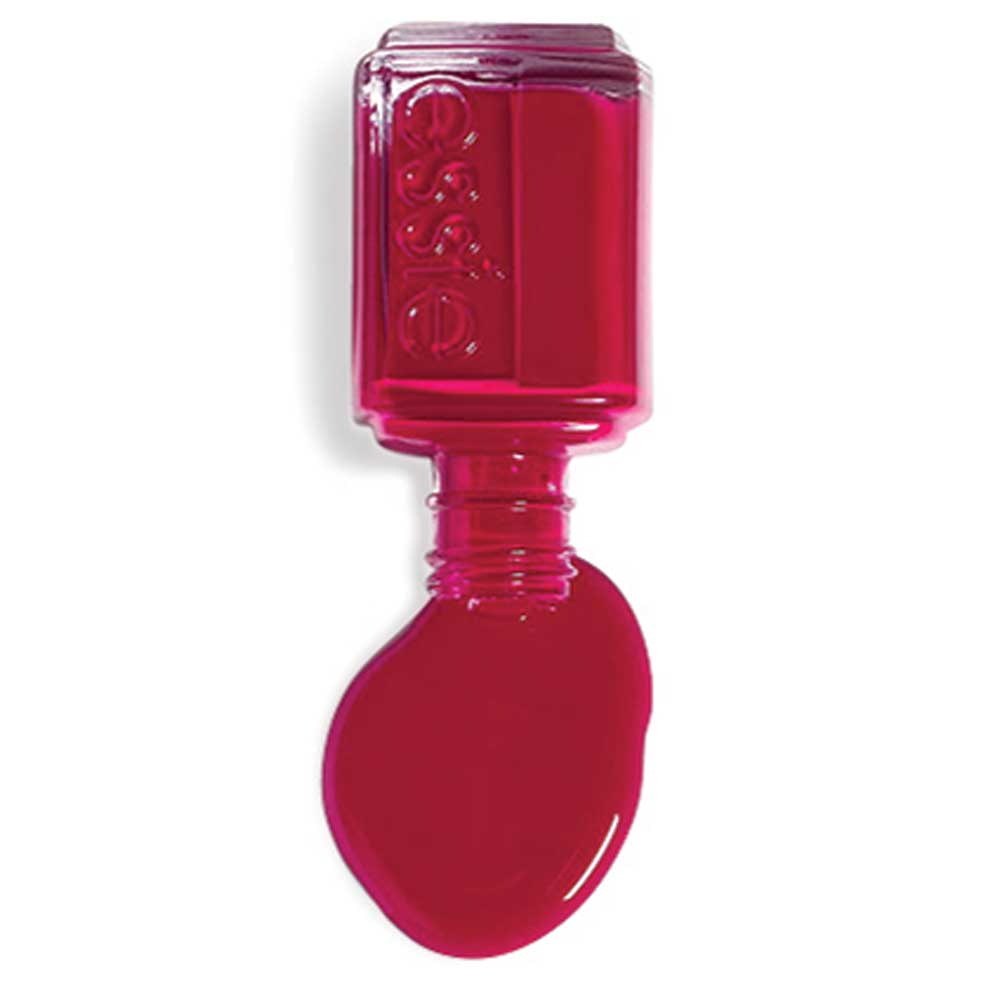The image depicts a small, clear glass bottle of Essie nail polish, approximately two inches in size, lying on its side, having spilled its contents. The deep maroon-burgundy nail polish, with hints of lavender and blood red, has formed a puddle on a solid white surface. The bottle itself is labeled "E-S-S-I-E" and has a light gray cast shadow to the left of the polished puddle. The intricate details of the spilled polish create a "lake-shaped" splatter, appearing darker than its contents due to a highlight area. The overall clean and minimalistic composition hints at an advertisement setting.